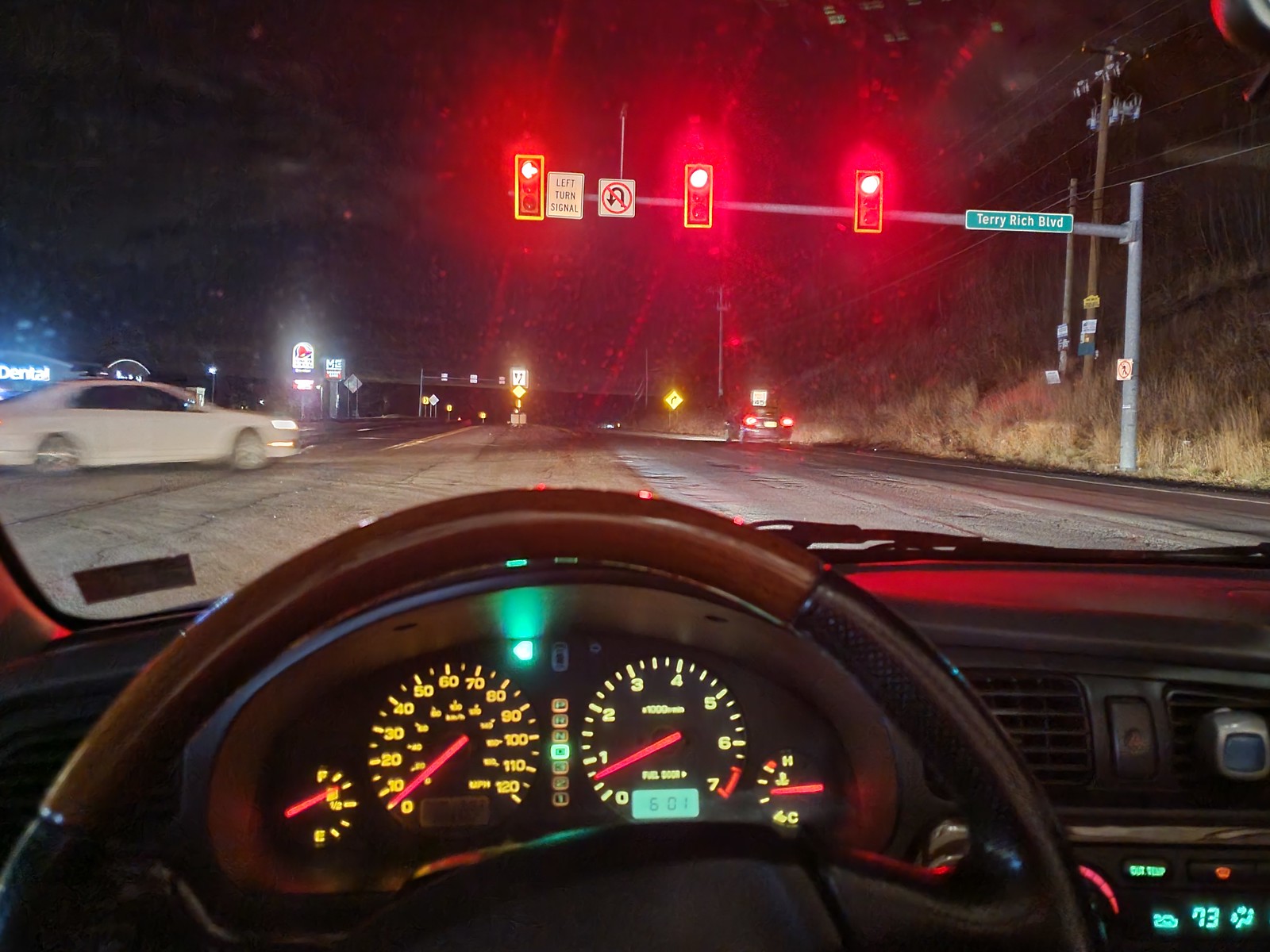From the driver's seat, this image showcases the car's black interior with a top half of the steering wheel in dark brown and black leather grips on either side. The dashboard features two large round dials for speed and RPMs flanked by smaller dials for fuel and radiator temperature, all with yellow indicators and red lines. Outside, the car is stopped at a traffic light with three signals, two of which are red and one showing a red arrow. Ahead, a rectangular green sign reads "Terry Rich Boulevard" atop a gray post. A white car is turning into the lane, and further down, a black car is parked on the right. On the right-hand side, there's a grassy hill. The scene is set at nighttime, with a Taco Bell visible in the distant background.